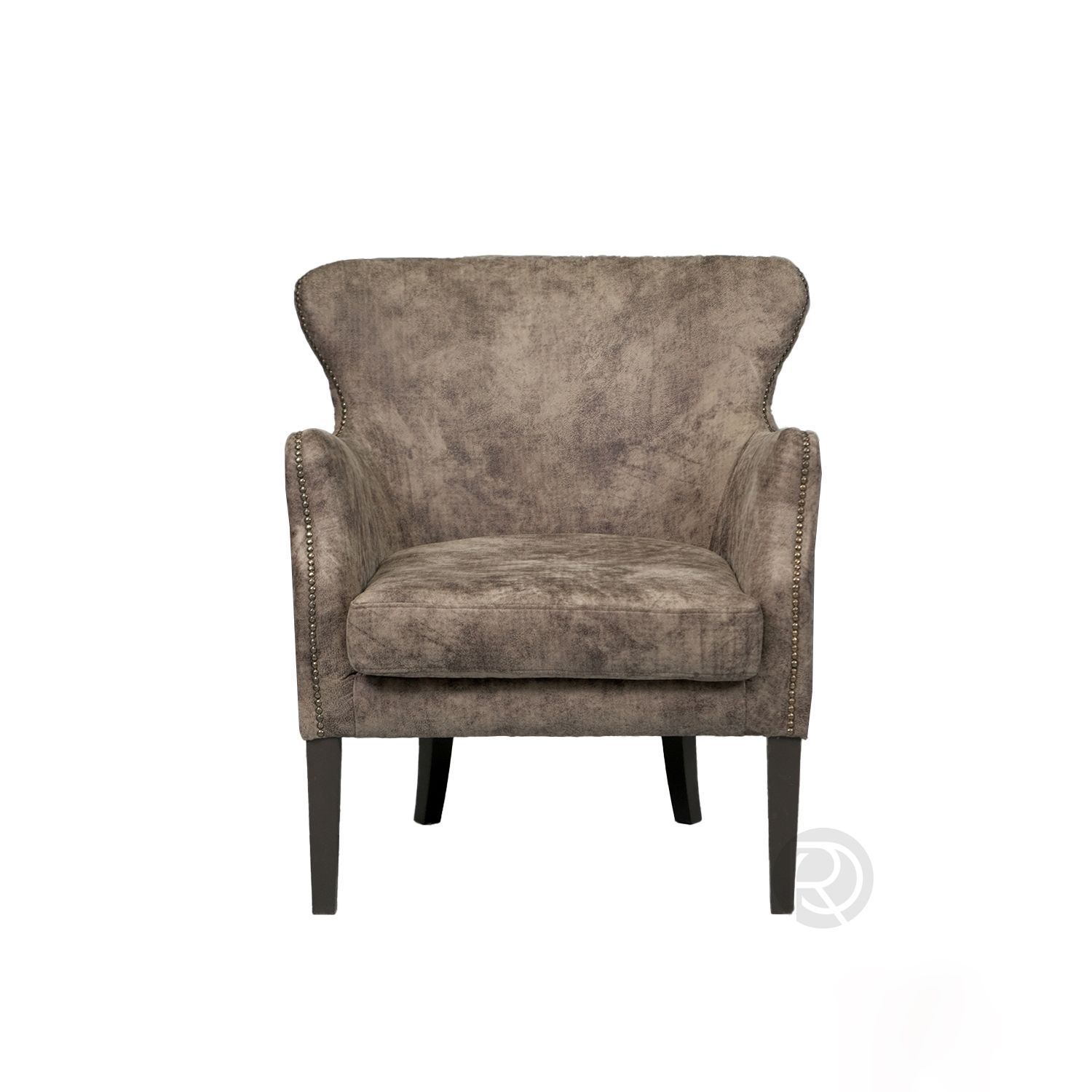The image showcases a Queen Anne-style chair positioned against a white background. This classic piece of furniture exhibits a two-tone blend of beige and light brown, almost appearing as mingled leather or suede. The wide back of the chair subtly flares outwards and is adorned with gold tacks along its edges and arms, providing a distinguished look. The back, although noticeably thick, doesn't feature a cushion but hints at a comfortable, foam-like structure. The seat cushion, matching the chair's material, looks plush and inviting. The chair stands on four dark wooden legs, with the front pair extending straight down and the back pair gracefully curving outwards. Despite its soft, cushioned appearance, the chair appears quite scuffed and dirty, possibly from wear and frequent use, giving it a lived-in, rustic charm.